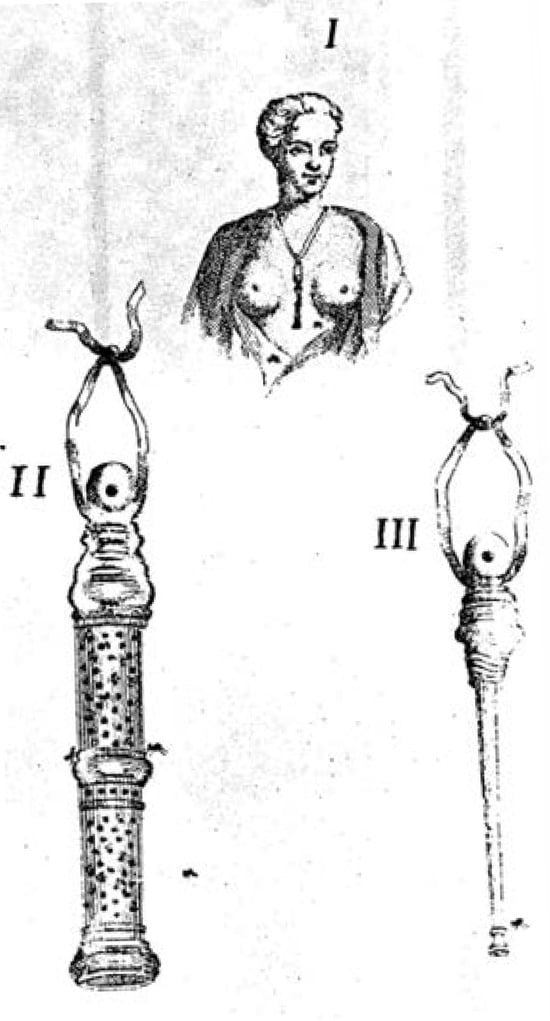This black and white historical drawing consists of three distinct sections, each labeled with Roman numerals I, II, and III. At the top, labeled "I," is a detailed illustration of a woman with her hair styled in a bun and her shirt open to expose her breasts. She is adorned with a prominent necklace. Below her, section "II" features an object resembling a column or pipe, which can be akin to a wooden musical instrument. This item is adorned with what appears to be a face with a mouth and a single eyeball, and has intertwined arms. The third section, "III," mirrors section "II," though it describes the object more like a long pendant with an eyeball in the center attached to a thin pole. These elements seem to provide a detailed and possibly symbolic depiction of the connections or steps relating to the woman and the items associated with her necklace.